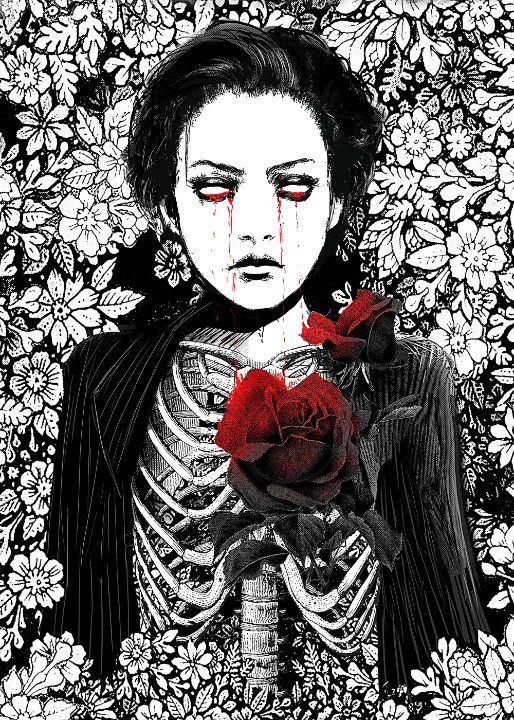The image is a dark, artistic drawing of a woman with a haunting, skeletal appearance. Her face is centered towards the top of the image, showing white, hollow eyes devoid of irises, from which blood red tears stream down. She wears a black, pinstriped jacket draped around her shoulders that reveals an exposed ribcage, detailed in stark black and white. Two red roses are prominently displayed in front of her skeletal midsection. The background contrasts sharply with its black base color, adorned with various black and white flowers and leaves, enhancing the eerie and twisted ambiance of the artwork. The overall composition and style suggest a fan-made piece, possibly created through silkscreen or oil painting techniques.